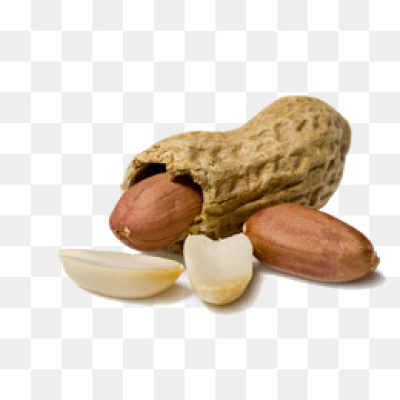This close-up image showcases a peanut with a white and gray checkerboard background commonly used in stock images to signify editable backgrounds. The central peanut shell is cracked open at one end, revealing a peanut partially protruding, still covered by its reddish-brown skin. Adjacent to the opened shell are three pieces of peanut meat: one intact with its brown skin on, and two broken pieces, stripped of their skin, displaying a creamy white interior with slight brown highlights. These elements are arranged prominently against the background, adding a graphical, almost surreal, quality to the image.